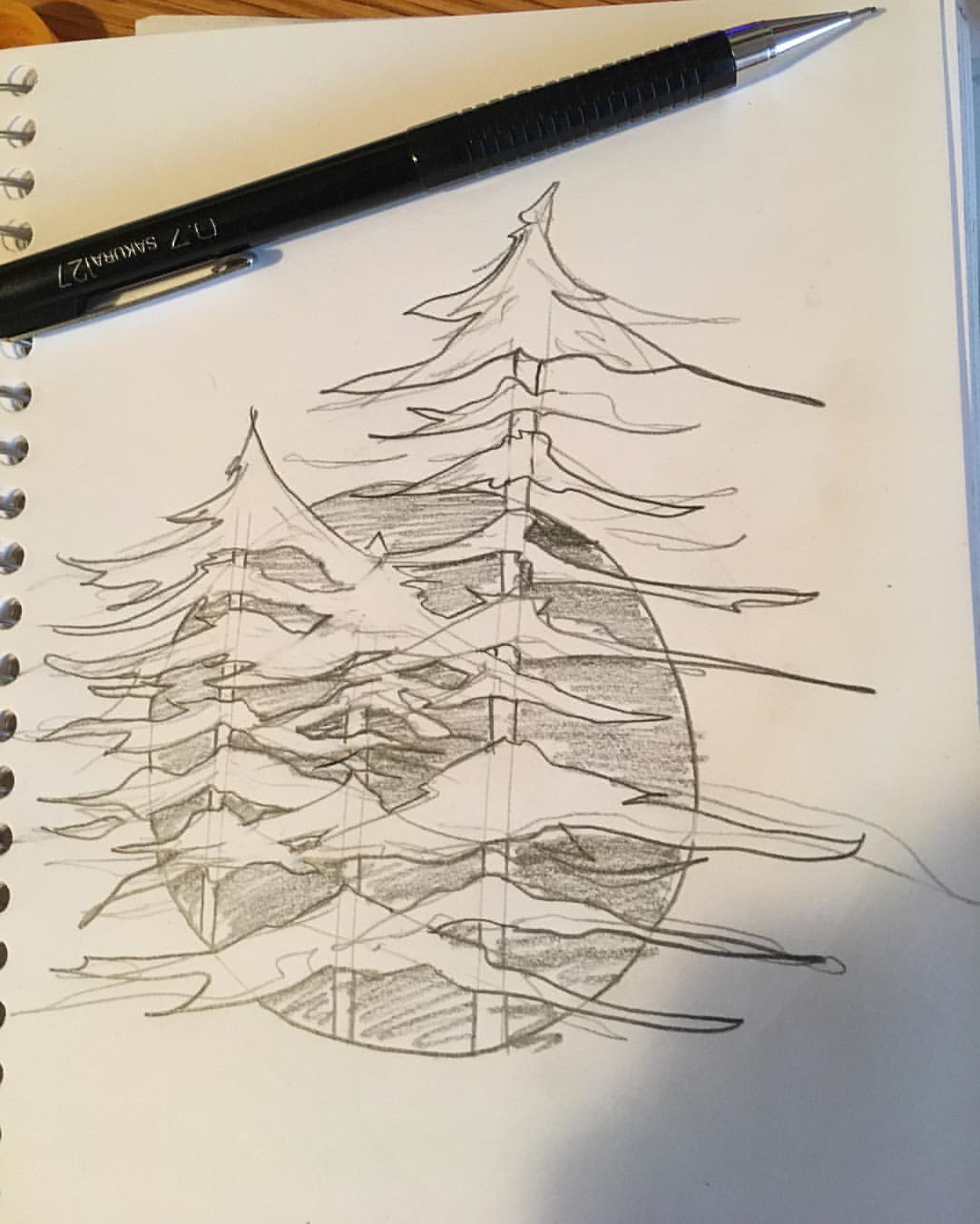The image showcases a page from a sketchbook, evident by the white paper and the silver-toned spiral rings along the left edge, threading through holes in the paper. The drawing appears to have been made with a mechanical pencil, which is also pictured at the top of the page. The mechanical pencil is black with a silver-toned tip, and a bit of lead is visible at its end, though the name written on it is illegible.

The sketch itself features a large gray circle, serving as a backdrop for three distinct trees. The tallest tree, situated on the right, extends well above the circle. To the left-hand side stands a medium-sized tree, while the third tree is slightly off-center to the left of the circle. These trees have unusual forms; their trunks are clearly visible from base to apex, with branches that extend outwards in a singular, elongated manner. They resemble pine trees in their overall shape.